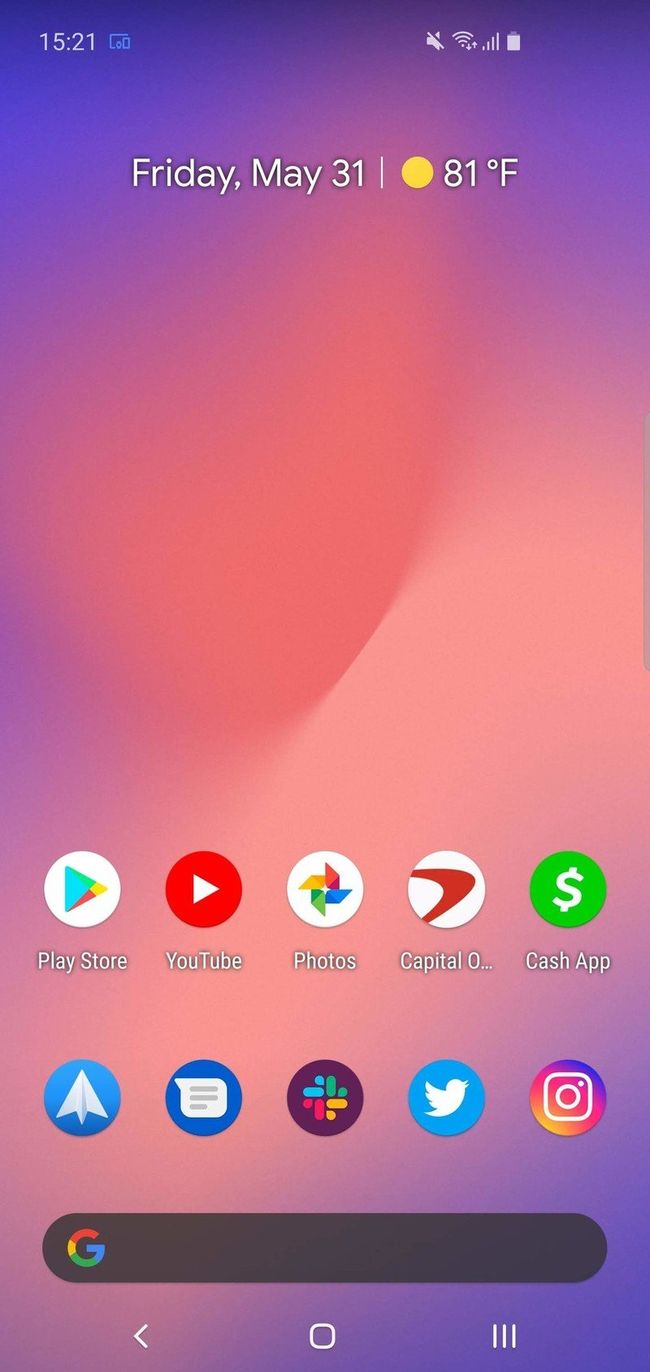This screenshot shows the interface of a cell phone. At the top left corner, the time is displayed as 15:21. Adjacent to the time, there's a small icon resembling a square with a rectangle beside it. On the upper right side, various status icons are visible: first, a speaker icon with a line through it indicating that the device is in silent mode, followed by the Wi-Fi signal icon and the cellular reception bars. The battery percentage icon is also shown. Directly below these icons, the date is displayed as "Friday, May 31st."

In the center of the screen, there is a weather widget featuring a yellow sun icon, indicating sunny weather and the temperature is shown as 81 degrees Fahrenheit.

Towards the bottom of the screen, there are several app icons neatly arranged: the Play Store icon, YouTube icon, Photos icon, and the Cash App icon. At the very bottom, the familiar Google search bar is prominently positioned. The overall layout and design suggest a typical Android device home screen, presenting essential information and frequently used apps at a glance.